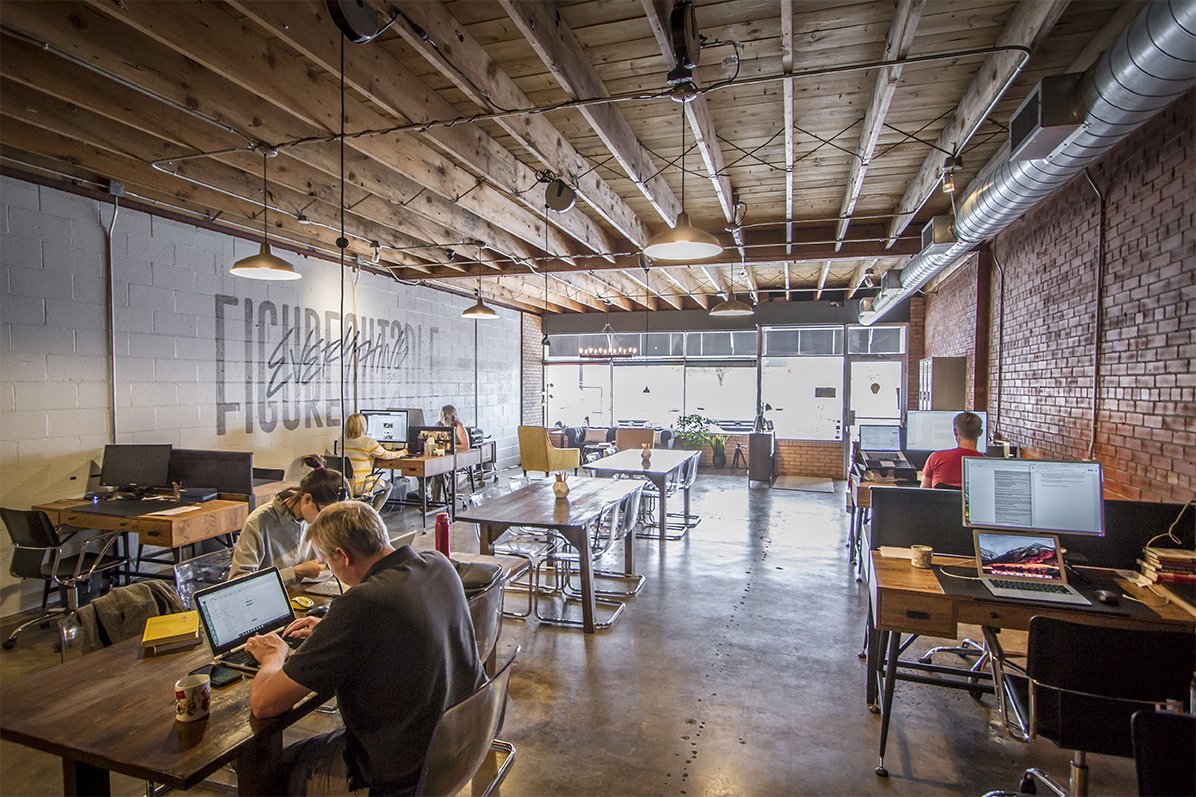This color photograph captures the inside of a transformed warehouse turned into a unique and cozy workspace. The warehouse features a raw aesthetic with a wooden beam ceiling adorned with hanging black metal lamps and running metal pipes. The walls vary, with the left side showcasing white cinder blocks and graffiti-covered writing, while a prominent red brick wall adds texture alongside. The polished cement floor reflects the soft, natural light streaming through large glass windows at the far end, indicating a bright, sunny day. The workspace is set with several wooden tables functioning as desks, each occupied by people working on computers. Notably, in the left portion, two women sit facing each other with desktop computers, while nearby, a man and woman work on laptops, though the man's head obscures the woman's face. To the right, a vacant desk displays both a laptop and a desktop setup. Wearing a red shirt, a man focused on his desktop computer sits somewhat centrally in the image. Overall, the muted yet vibrant colors, graffiti details, and informal layout create an inviting, productive atmosphere.